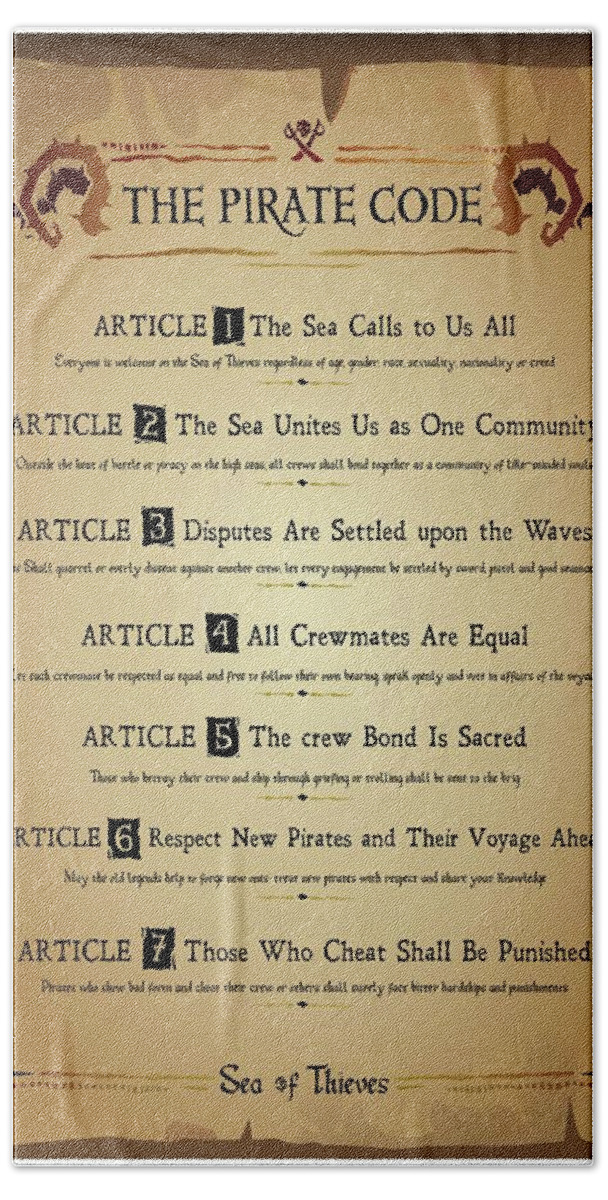This image depicts a wrinkled, beige poster with an aged appearance, featuring an old-fashioned font. At the top, in the middle of a dark brown, irregular border, is the title "The Pirate Code," accompanied by a small skull and crossed swords icon just above it. Below the title, the poster is organized into seven articles, each followed by an illegible line of tiny print. 

The articles are as follows:
1. The sea calls to us all.
2. The sea unites us as one community.
3. Disputes are settled upon the waves.
4. All crewmates are equal.
5. The crew bond is sacred.
6. Respect new pirates and their voyage ahead.
7. Those who cheat shall be punished.

At the very bottom of the poster, just above another portion of the irregular dark brown border, the text reads "Sea of Thieves."